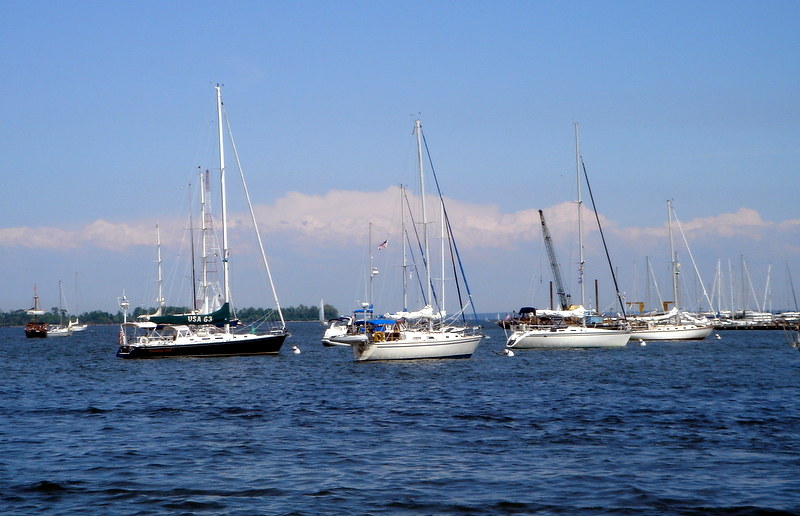In this detailed rectangular photograph, set in a landscape orientation, we see a serene waterway under a vibrant blue sky peppered with wispy white clouds. The dark blue water is calm with gentle ripples, suggesting a mild breeze. The image prominently features approximately a dozen sailboats anchored, their white hulls and masts creating a striking contrast against the dark water.

A notable sailboat on the far left stands out with its blue hull and the inscription "USA 63" on its flag area. The rest of the sailboats have white hulls, with some boats to the right showing dark blue or black accents on their secondary masts, while their main masts remain white. None of the boats have their sails out, as they are all furled.

In the distance to the left, smaller sailboats can be observed, clustered together towards a wooded shoreline. This wooded area, featuring tall trees with dark green leaves, juts out into the water and provides a natural backdrop. The pleasant weather and gentle waves emphasize the tranquility and beauty of the scene.